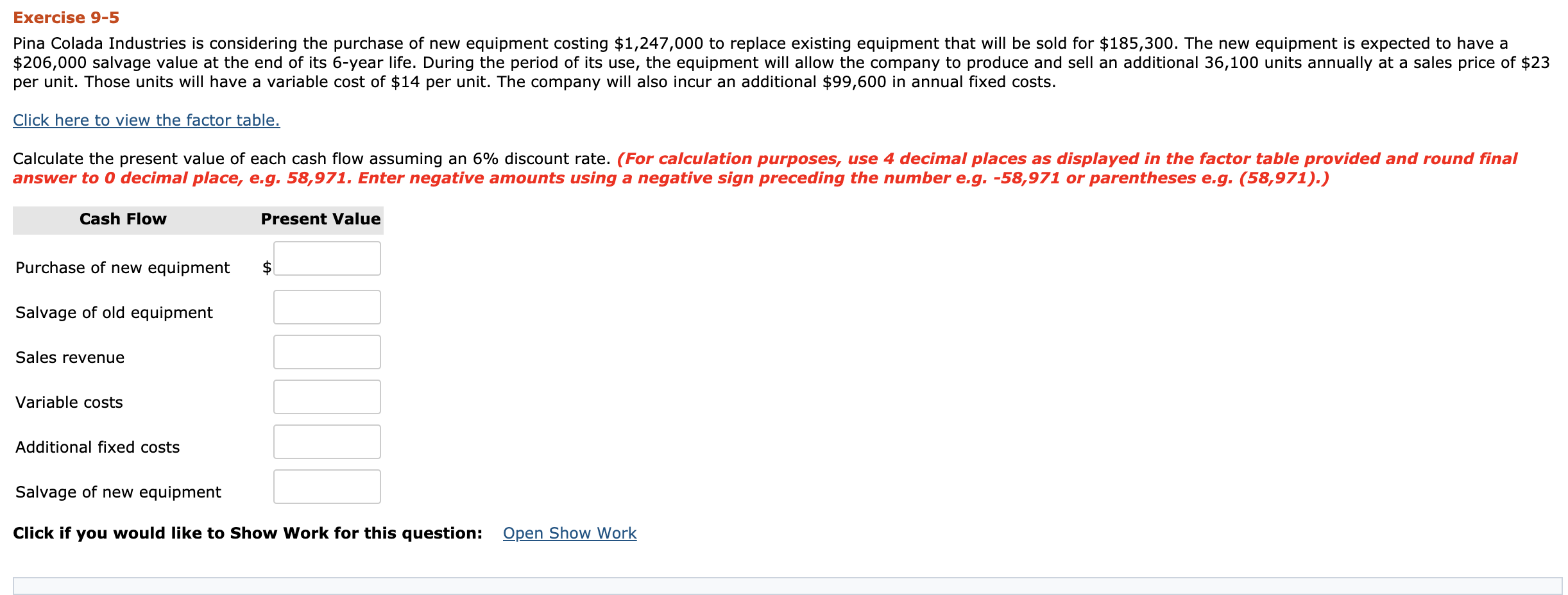**Detailed Descriptive Caption:**

"Exercise 9-5 from an accounting class requires evaluating the financial decision of Pina Colada Industries regarding the acquisition of new equipment. The scenario involves purchasing new equipment for $1,247,000, which will replace the old equipment that can be sold for $185,300. The new equipment is projected to have a salvage value of $206,000 after its 6-year lifespan. Furthermore, it is expected to increase the production capacity of the company by 36,100 units per year, with each unit selling at $23 and incurring a variable cost of $40. Additionally, the company will face an increase in annual fixed costs by $99,600. The task includes calculating the present value of each cash flow using a 6% discount rate, with cash flow categories and corresponding present value inputs outlined (Purchase of New Equipment, Salvage of Old Equipment, Sales Revenue, Variable Costs, Additional Fixed Costs, Salvage of New Equipment). Calculation instructions specify the use of four decimal places for factors and rounding the final answers to zero decimal places, with negative amounts indicated by a preceding negative sign. The exercise provides a layout for entering cash flows and their present values along with an option to view detailed work via a "Show Work" feature."